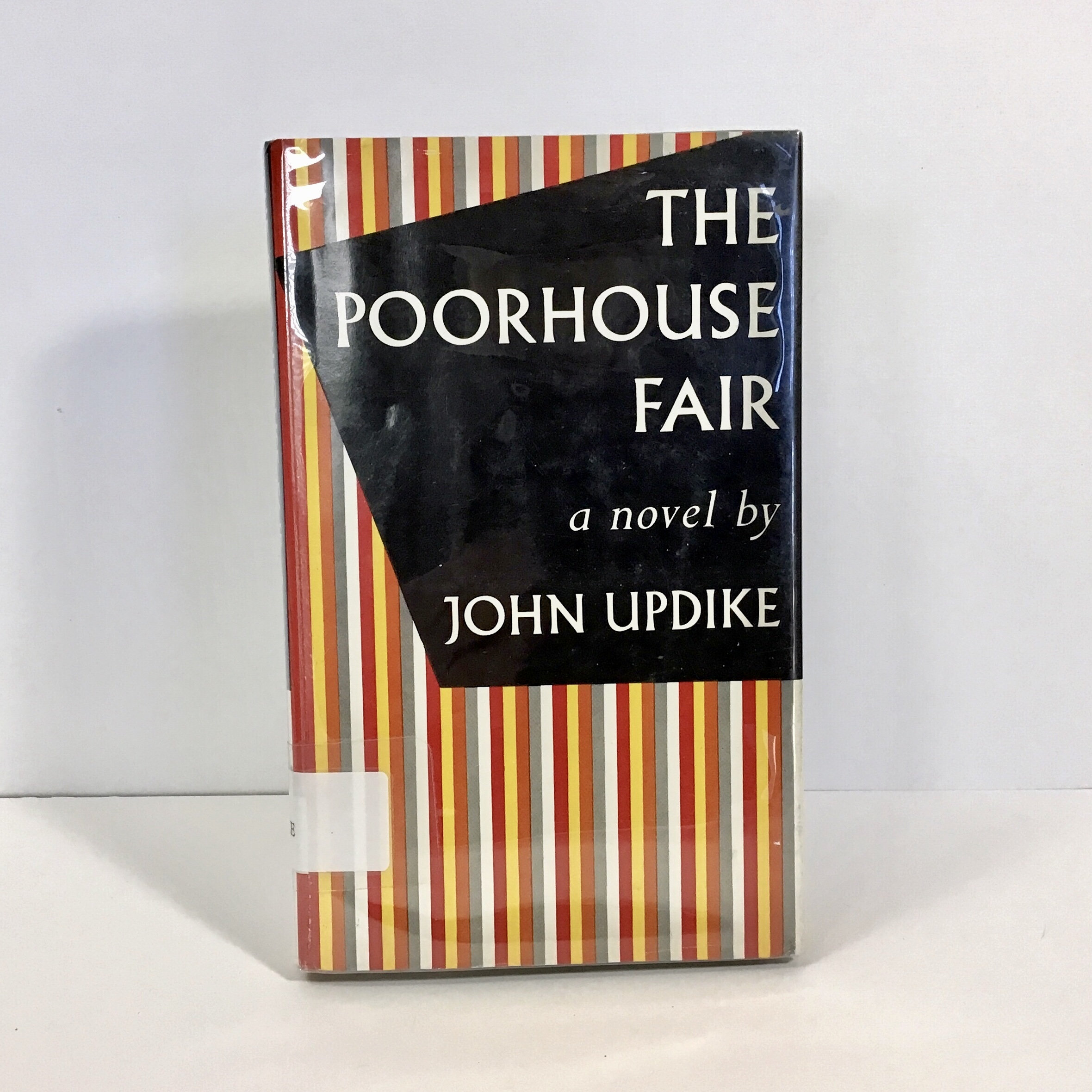The image depicts a hardcover book titled "The Poor House Fair, a Novel by John Updike." The cover design is minimalistic, featuring vertical stripes in a repeating pattern of red, orange, yellow, gray, white, and beige. The stripes span the entire surface of the book, creating a somewhat monotonous visual effect. The book title and author’s name are prominently displayed in a serif-style font that contrasts with the vivid stripes. There is a small white section at the bottom of the cover, possibly containing library or ISBN numbers. The photograph appears to have been taken in a well-lit studio or home setting, with the book placed on a white background, highlighting its simple yet striking design.